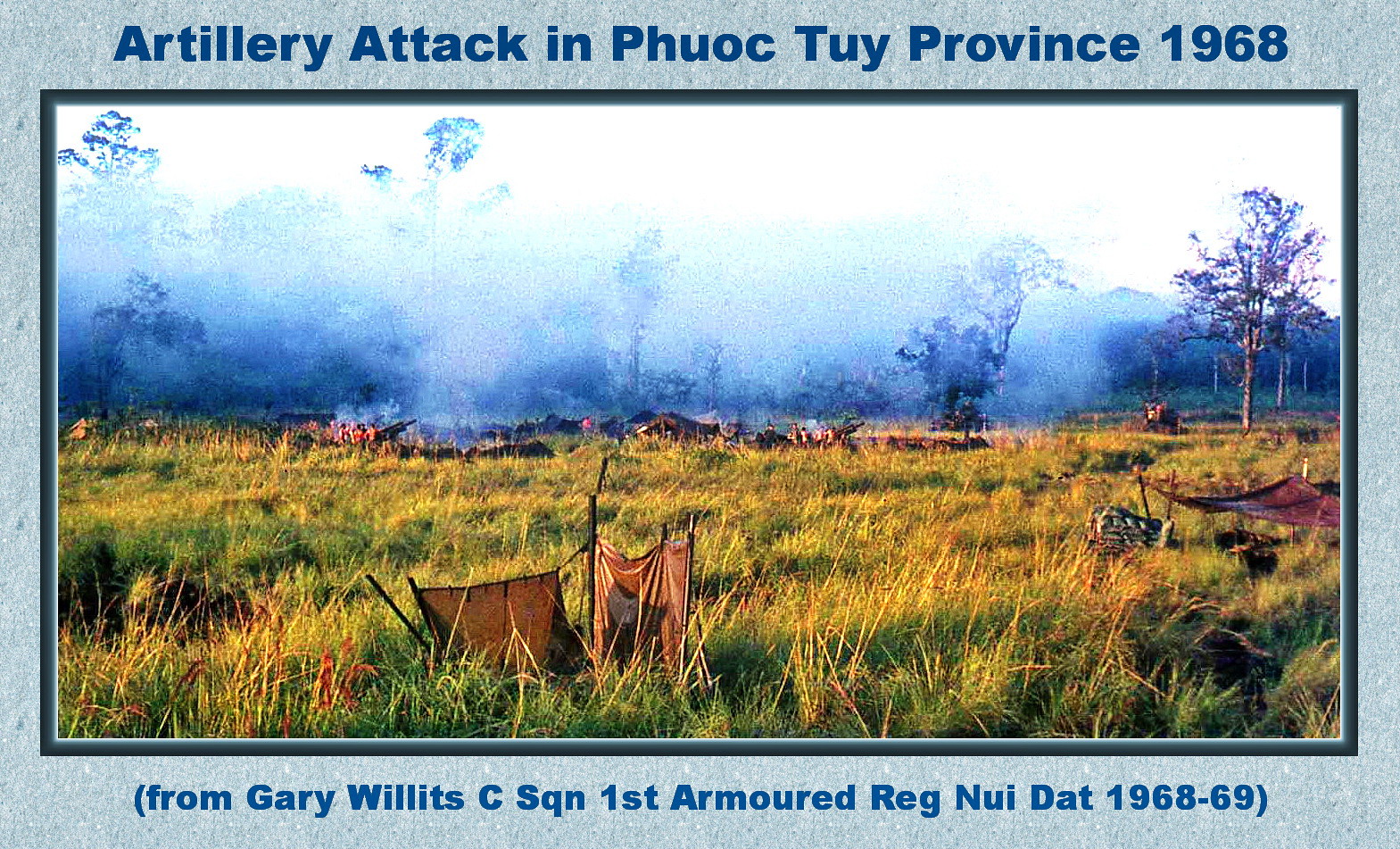This vintage or recreated photograph captures a scene of an artillery attack in Fyoktoy (or Bauk, Thai) Province, dated 1968. The image is framed by a border and features a dramatic backdrop of smoky haze and visible, though somewhat obscured, trees due to the smoke. The sky is a pale white, blending into the smoke coming from the flames in the background. The foreground is dominated by an overgrown field of green and yellow grass. On the right side of the photograph, a red hammock is noticeable, while to the left, a yellow tarp-like material is suspended by dark-colored sticks or bars. The scene is framed with a gray or black outline.

The photograph's colors prominently include shades of green, yellow, blue, white, and smoky greys. At the top of the image, an inscription in dark blue font on a lighter blue background reads "Artillery Attack in Fyoktoy Province, 1968" (with variations noted). Beneath the picture, a similar blue font on a slightly different shade of blue background states, "(From Gary Willis C. SQN, 1st Armored Reg, Mui Dat, 1968-1969)" or "(From Gary Willits, C.S.Q.N. First Armored Reg, Naui Dat, 1968-69)". This caption signifies that the image is a documented memory or reimagined depiction of a historical military event from 1968.